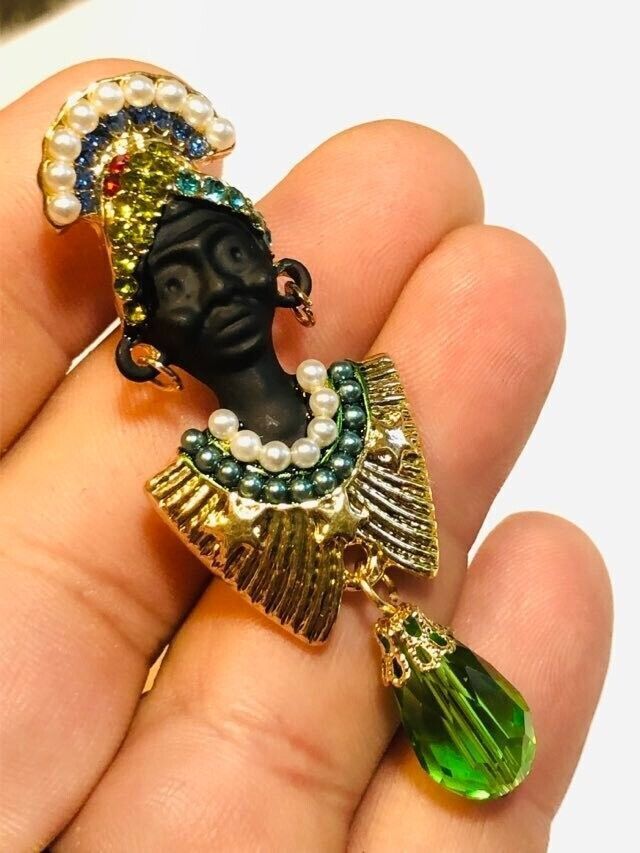In this close-up photograph, a fair-skinned individual's left hand is delicately holding an ornate pin that depicts an African woman adorned with an array of vibrant jewels. The detailed image showcases the person's four fingers, with visible fingerprints against a predominantly white background, interrupted by a small brown blur in the top left corner. The African woman on the pin is carved in deep black, possibly ebony, and she is elegantly decorated with a gold and jewel headdress featuring pearls at the top. The headdress and jewelry include vibrant gems in gold, red, blue, and turquoise. She wears small gold hoop earrings through notably large ear piercings, a pearl necklace, and another beaded necklace underneath. Her figure elegantly tapers into a gold V-shape, and a striking green gem is suspended at the bottom of the pin, accentuating the intricate craftsmanship of this miniature piece of jewelry.